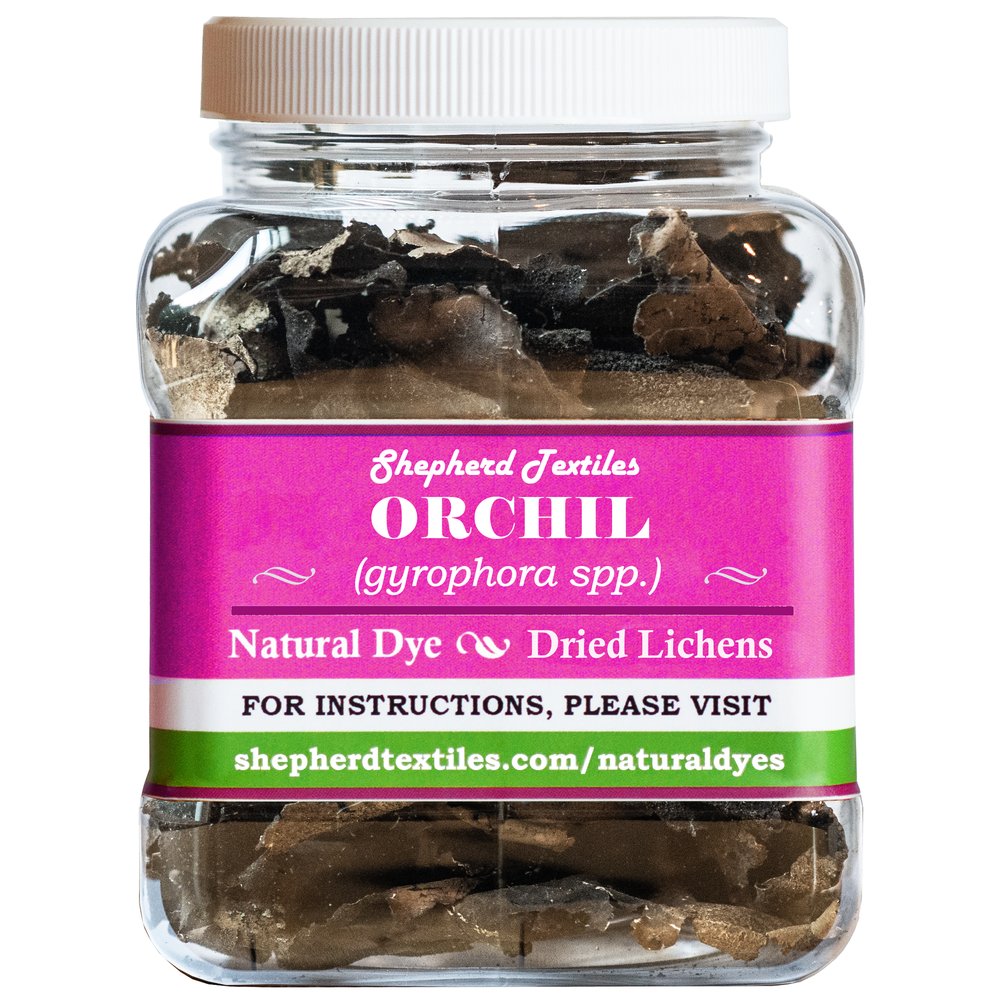The photograph showcases a square-shaped jar made of clear acrylic or plastic, revealing its brown, leafy, dried contents, which appear to be dried lichens. The jar is completely full and features a white, screw-top lid. It is presented against a flat white surface and background, ensuring the focus remains solely on the product. The jar is adorned with a prominently placed label that spans the center of the jar. The label is primarily pink at the top, transitioning to white in the middle, and green at the bottom. The label reads: "Shepherd Textiles, Orchil, Gyrophora SPP (Natural Dye Dried Lichens)." For further instructions, it directs users to visit "shepherdtextiles.com/natural dyes."